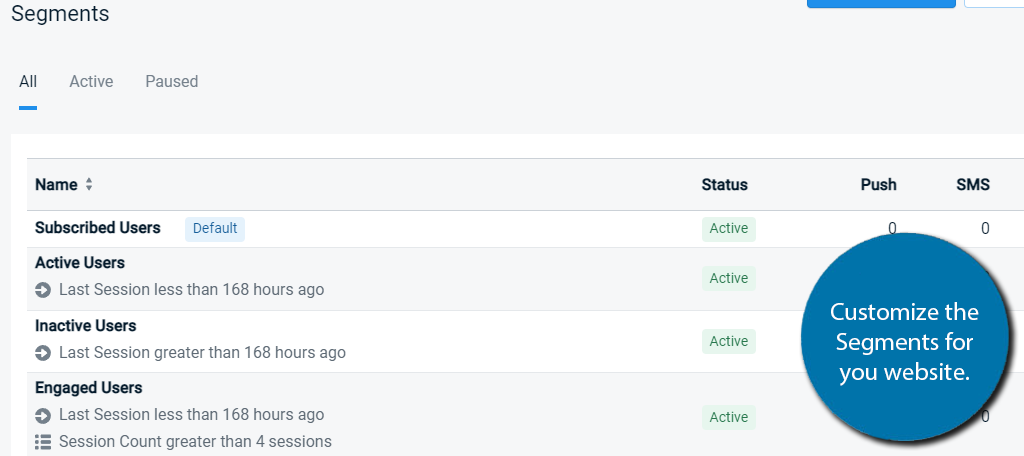**Detailed Caption:**

The image appears to be a screenshot showcasing the functionality of a webpage segment customization feature. At the top of the page, there's a grey box with dark grey text, highlighting different segment views. Just beneath this box, there are three filter options: "All", "Active", and "Paused". The "All" filter, underlined in blue, is currently selected.

Below the filters, there's a white table divided into several columns: *Name*, *Status*, *Push*, and *SMS*. The table has multiple rows detailing various user segments:

1. **Subscribed Users**
   - Status: Active
   - Push: 0
   - SMS: 0

2. **Active Users**
   - Last session: Less than 168 hours ago
   - Status: Active

(Note: Some information is obstructed by a circle overlaid on the table.)

3. **Inactive Users**
   - Last session: Greater than 168 hours ago
   - Status: Active

4. **Engaged Users**
   - Last session: Less than 168 hours ago
   - Session count: Greater than 4 sessions
   - Status: Active

Also, obscured details involve Push and SMS specifications for the engaged users. 

Covering part of the table in the bottom right corner, there is a blue circle with white text that reads: "Customize the segments for your website." This circle is likely a call-to-action or an informational tooltip, emphasizing the feature's purpose of segment customization for the site.